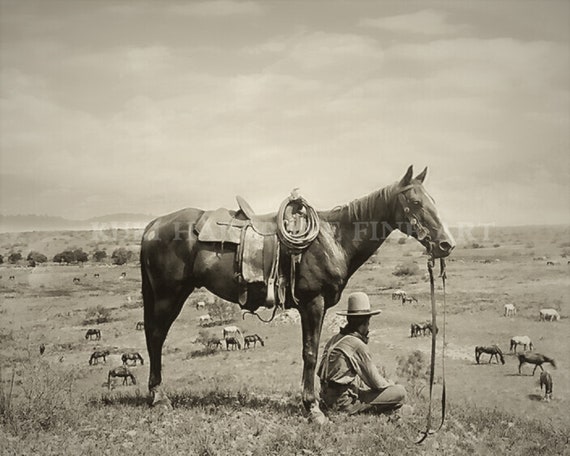This vintage black-and-white photograph, marked with a semi-transparent "Kith Heart Fine Art" watermark at its center, captures a tranquil scene atop a hill. In the foreground, a man sits cross-legged, dressed in long pants with suspenders crossing on his back, and a long-sleeved button-up shirt with a collar, complemented by a bandana around his neck. He wears a round-top cowboy hat adorned with a dark-colored band. Behind him, a horse stands with its reins laid on the ground beside the man. The horse is equipped with a leather saddle and a coiled rope around the saddle pommel. The background features a sweeping view of a valley dotted with over a dozen grazing horses of varying colors. The top half of the image shows a skyline rendered in a light brownish-gray hue with faint, almost indistinguishable clouds. The serene openness of the field extends to the horizon where a few scattered trees and distant mountains blend into the grayscale vista.